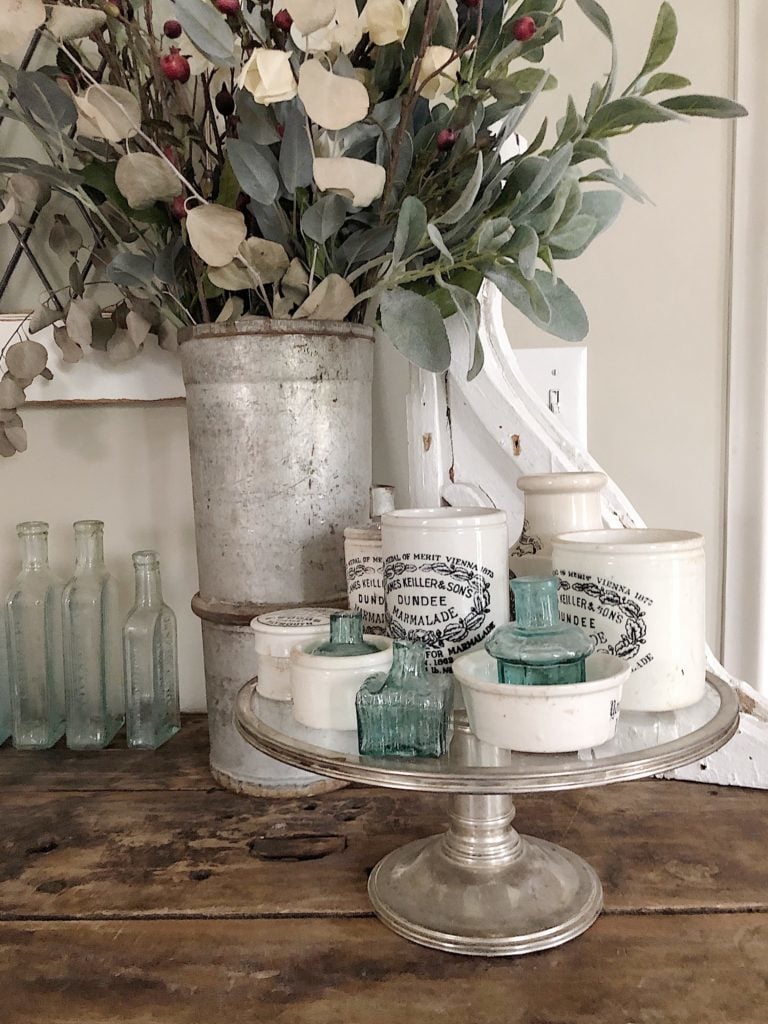The image captures a visually striking vignette blending vintage and modern elements. It features a distressed wooden table with visible seams and black stains that give it an aged appearance. The pristine, light gray or cream-colored wall with white trim in the background, along with a modern light switch, suggests a contemporary setting. On the left side of the table, three vintage-looking, square glass bottles are neatly lined up, with two being taller and one medium-sized. A cylindrical metal vase holds a mixture of light green and white leaves, along with a few red berries and dried eucalyptus branches. Positioned centrally towards the right and bottom of the image is a metal tray with a mirrored top, displaying several white cylindrical containers labeled “James Keller and Sons Dundee Marmalade.” Among these containers are three green-tinted glass bottles, two of which are nestled within the jars. The overall color scheme features a harmonious blend of whites, silvers, greens, and blues, creating a nostalgic yet stylish display.